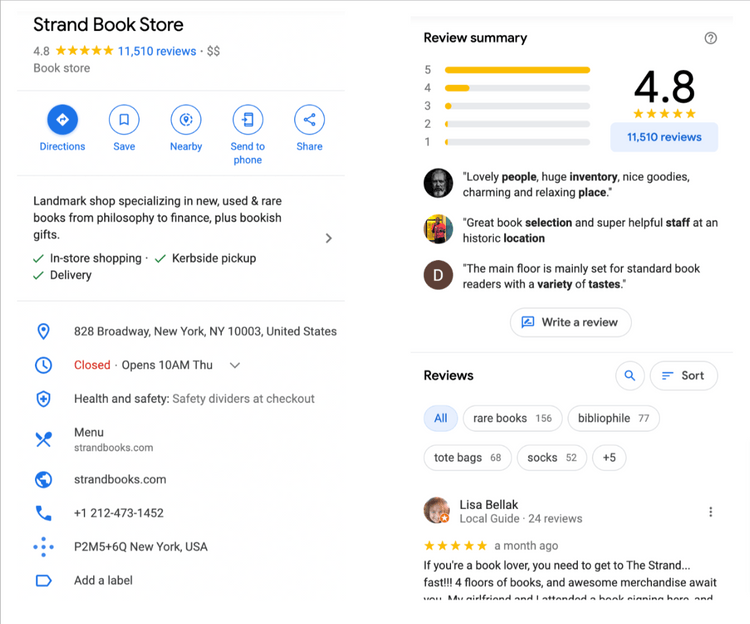The image displays a detailed overview of the Google reviews for a bookstore. At the top left corner, there is a very thin grey bar that partly forms a square but isn’t fully visible. 

On the left-hand side, the business name, "Strand Bookstore," is prominently displayed against a white background. Adjacent to this, the bookstore boasts an impressive 4.8 rating out of 5 stars, with the stars highlighted in gold and viewed by 11,510 reviewers, indicated in blue text. The price range, denoted by two dollar signs in grey, is listed just below, followed by the category tag "Bookstore."

There are five interactive blue buttons below this: 'Directions,' 'Save,' 'Nearby,' 'Send to Phone,' and 'Share.' The 'Directions' button has a more shaded blue background compared to the others.

Below the buttons, black text provides a description of the bookstore as a "Landmark shop specializing in new, used, and rare books in philosophy and finance, plus bookish gifts." Additional services include in-store shopping, curbside pickup, and delivery options.

The bookstore's address is listed as "828 Broadway, New York, NY 10003, United States," accompanied by its opening hours, noting that it’s currently closed but will open on Thursday at 10 am. Information about safety measures, particularly safety dividers at checkout, is also mentioned. The store's website, strandedbooks.com, and its contact number, +1-212-473-1452, are provided.

On the right-hand side of the image, there are review summaries highlighting the overall 4.8 ratings, with details on how many 5-star, 4-star, 3-star, 2-star, and 1-star reviews the store has received. Additionally, there are some selected quotes from customer reviews.